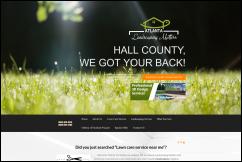The image appears to be a compact, blurry screenshot from a website. The upper part of the image features a black section with sunlight rays filtering through, and beneath that, there is grass. Towards the left edge, a gap in the black section reveals some green and white elements. 

There's a distinctive white icon that could be interpreted either as a cloud, a fish, or a house with a small hand-like detail, reminiscent of a teapot. Adjacent to this icon is white text stating "Hale County, we've got your back." 

Further down, the content includes a mix of bands and rectangles in varying colors: a black band with white text, a white band with black text, and an orange rectangle with yellow text. Below the “Hale County” slogan, there is a visually indistinct orange rectangle that seems to contain an image of a swimming pool and some trees, making it difficult to discern. 

On the left-hand side, green and white text is visible, though unreadable. The black and white bands feature text that remains too pixelated to decipher even when zoomed in. Despite the visual fragments, the context suggests the image may promote some type of property or property development, though the details are largely obscured by its diminutive size and lack of clarity.